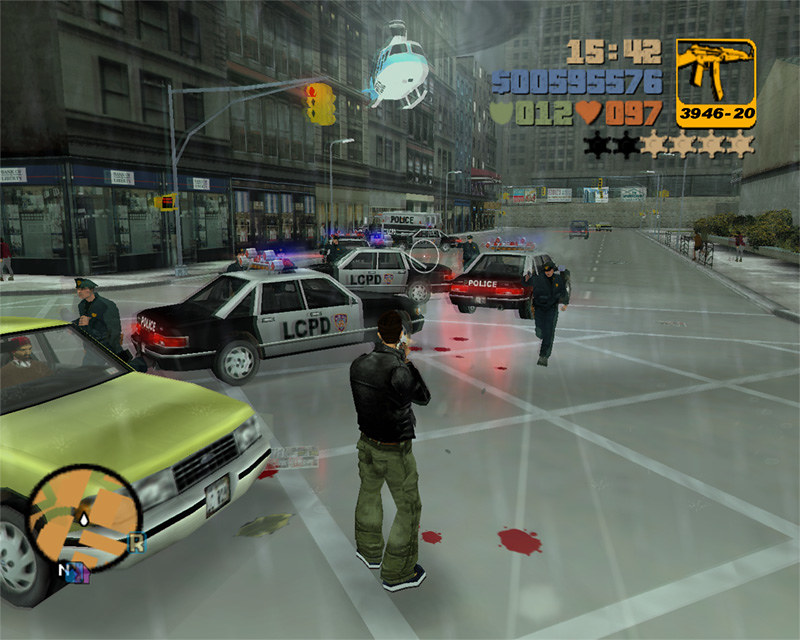This screenshot, likely from an early Grand Theft Auto game such as GTA 3 or San Andreas, captures a moment of intense chaos in an urban intersection. The graphics are notably pixelated, reflective of early Playstation and console eras. Central in the image, the main character stands amidst the turmoil, equipped with a machine gun boasting exactly 3,946 bullets. The character's status is displayed in the upper right corner: a time of 1542, a substantial wealth of $595,576, 12 armor points, 97 health points, and a high wanted level of 4 out of 6 stars. Surrounding him are seven police cars and five officers, with a helicopter looming overhead, signaling escalating law enforcement response. Additional details include a yellow card in the bottom left-hand corner and a mini-map, enhancing the tactical aesthetic. Distinctive elements like a person walking down the right side of the street and multiple cars in the backdrop amplify the scene's frenetic energy and realism. Bloodstains on the ground hint at the recent violence and the dire situation as the protagonist navigates the virtual cityscape.